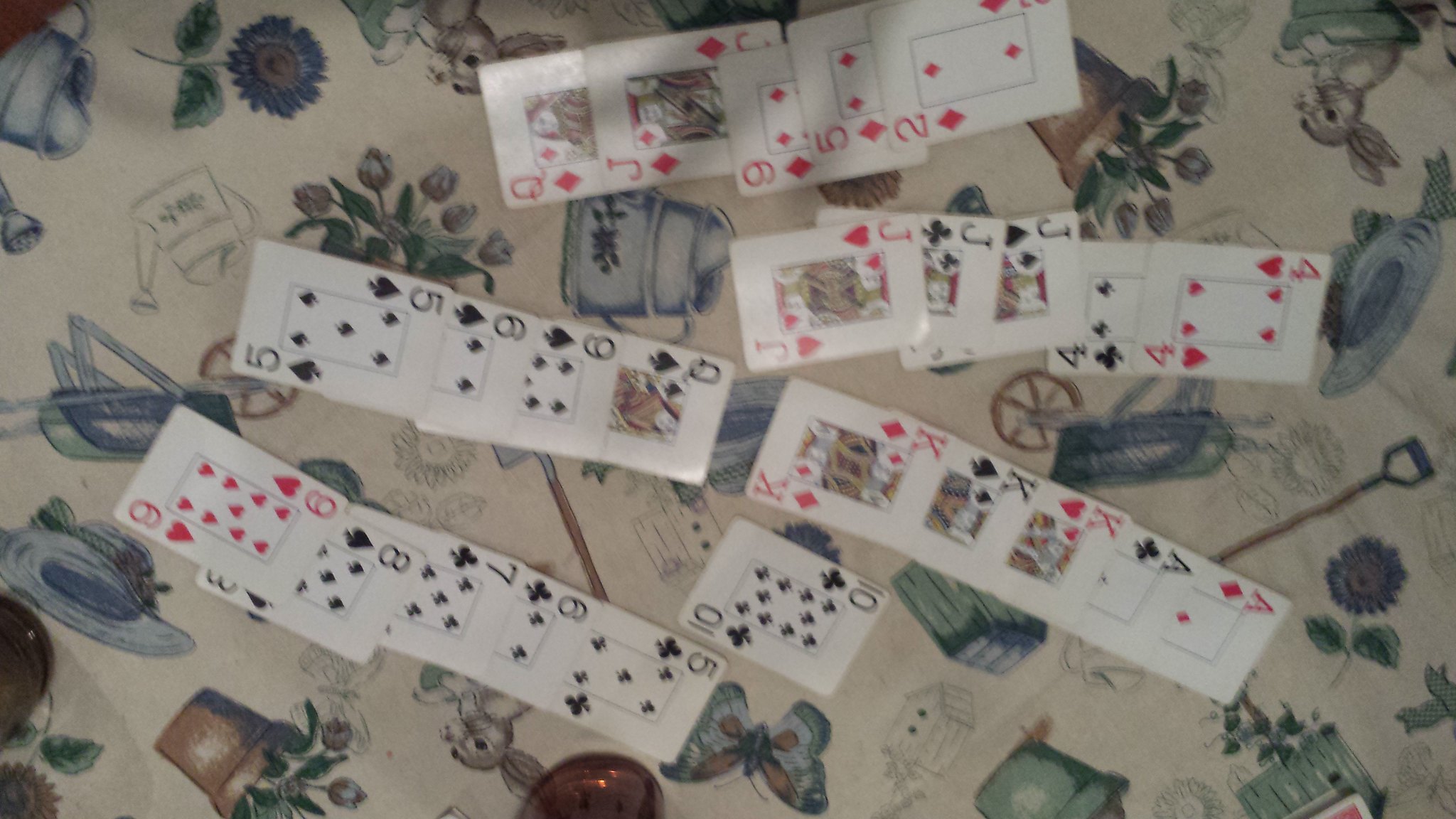This overhead color photograph captures a clutter of playing cards arranged on a patterned tablecloth. The cards, notable for their large, wide type, are laid out in various stacks. Dominating the top of the scene is a pile featuring the Queen, Jack, Nine, Five, and Two of Diamonds. Slightly to the right and below this is another stack displaying the Jack of Hearts, Jack of Clubs, Jack of Spades, Four of Clubs, and Four of Hearts. Positioned to the left of center is a grouping with the Queen, Nine, Six, and Five of Spades.

To the right of these cards and aligned vertically are a sequence of three Kings and two Aces. Directly underneath this vertical line is a solitary Ten of Clubs. Spread out from this pile towards the left side are the Five of Clubs, Six of Clubs, Seven of Clubs, Eight of Spades, and Nine of Hearts, forming a linear arrangement. 

The off-white tablecloth beneath the cards features a delicate pattern of kettles and pastel-colored flowers and plants in hues of blue, brown, and pink. The overall image is slightly blurry and out of focus, adding a soft, atmospheric quality to the scene.